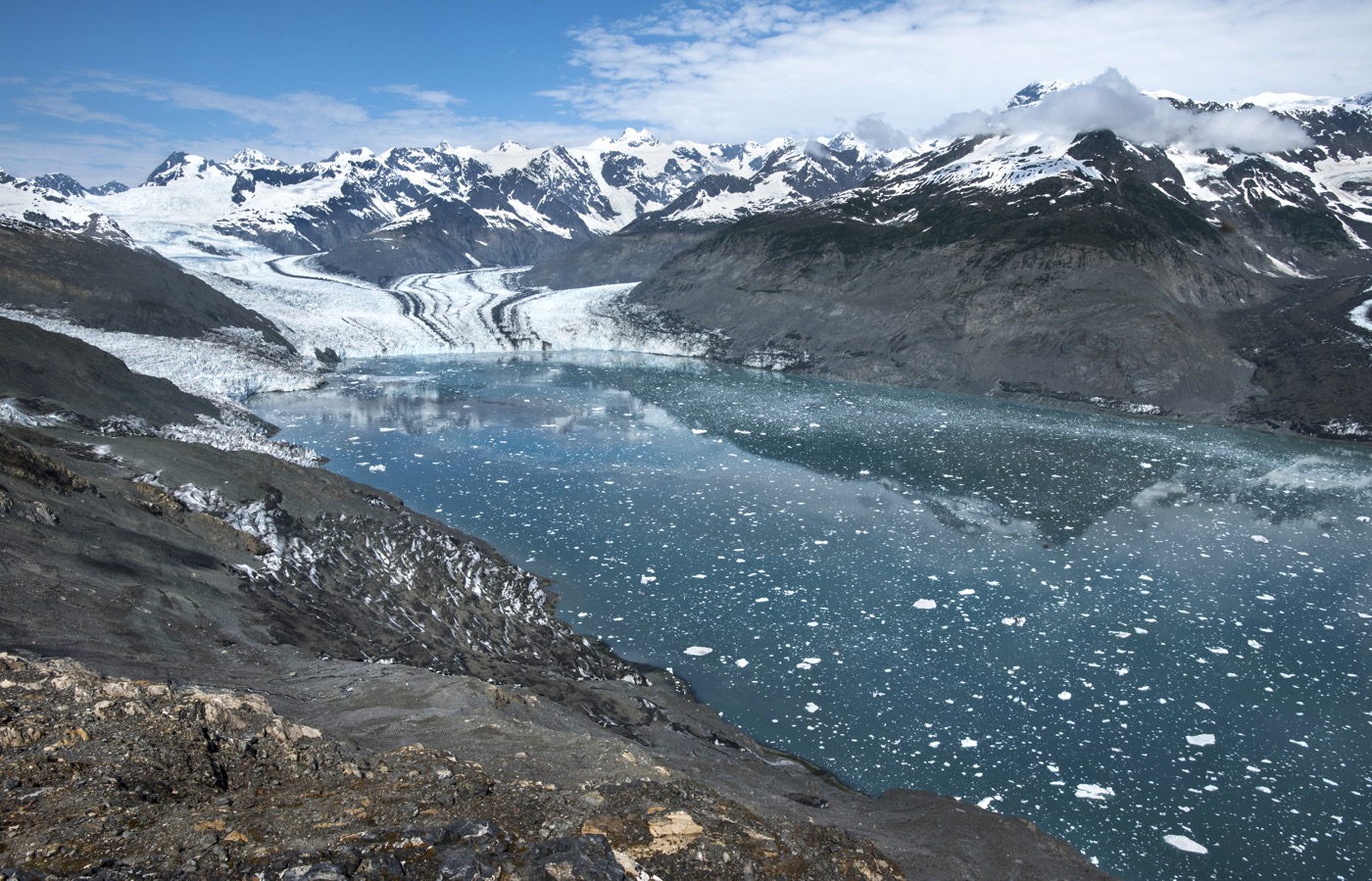The photograph is a captivating landscape showcasing a large mountain lake, which dominates roughly half the image. The lake's water is a striking, luscious blue-green, transparent and highly reflective, mirroring the surrounding rugged mountains and sky. Several ice floes speckle the surface, hinting at the waning days of winter, yet the cold still grips the scene. Encircling the lake are towering, craggy mountains capped with snow, their peaks reaching into the sky. In the background, some sharp, snow-covered peaks merge with wispy clouds and patches of blue sky. A puffy cloud lazily floats lower than some of the highest summits. The foreground on the bottom left features bare stone with sparse snow coverage and hints of moss and lichen. Near the upper left, faint tracks suggest a vehicle might have traversed the desolate landscape recently. The overall scene is one of serene, cold beauty, evocative of a high-altitude wilderness in the late stages of winter thaw.